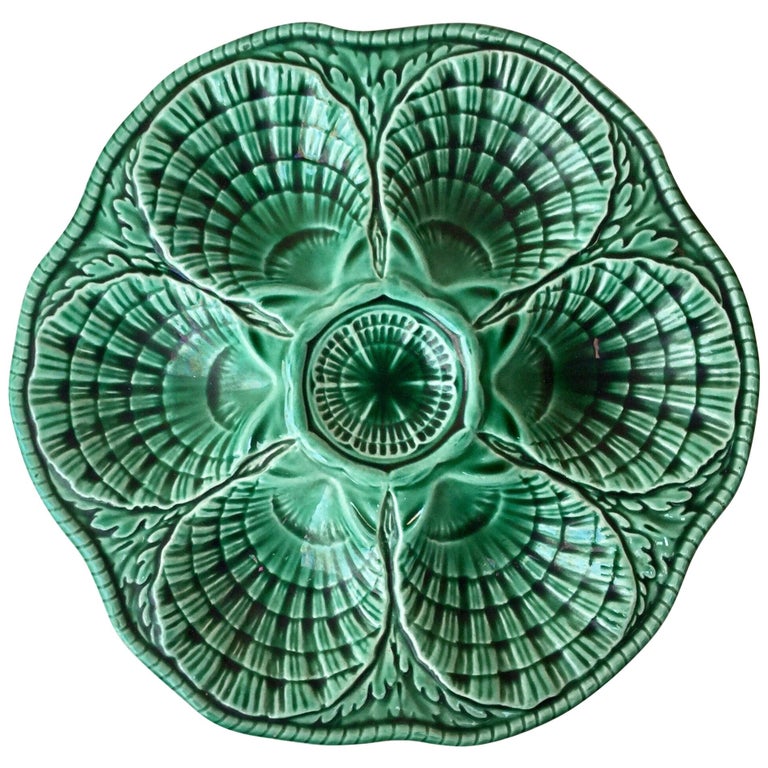This image depicts a highly decorated jade-green ceramic plate viewed from the top down, with the background removed for a clear focus on the object. The plate, resembling a piece of artwork, features six scalloped, shell-like sections radiating around a hollow central area. These sections, which could serve for placing different appetizers or sauces, exhibit intricate leaf patterns and darker green grooves. The plate’s outer edge is adorned with a delicate, thin striped border, adding to its elegance. The overall design and coloration suggest a harmonious blend of light and dark greens, making it not only functional but also visually appealing, potentially as a serving dish or an ornate decorative piece.